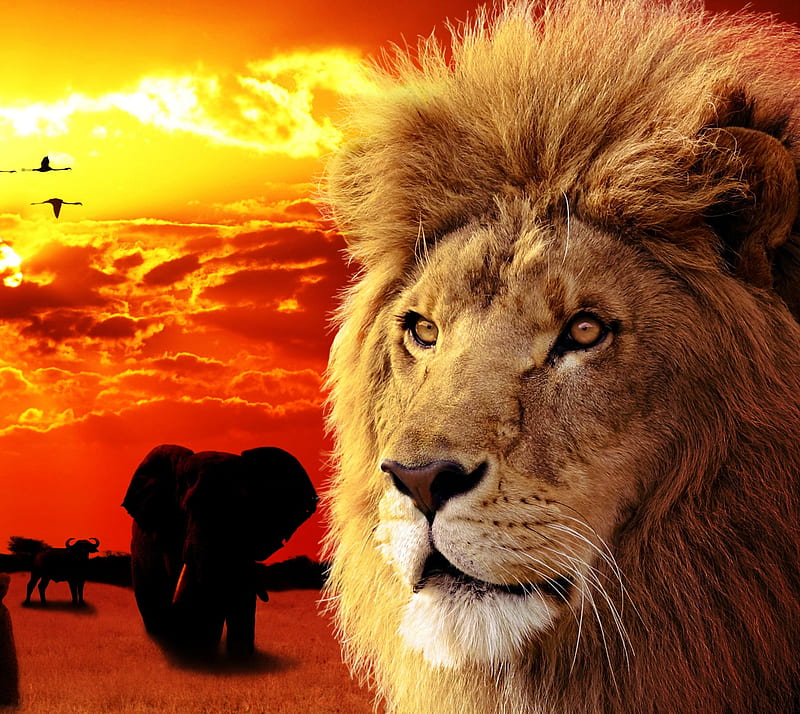This vivid image captures the intense intimacy of a lion's face, its thick mane framing brown fur and white around its mouth, set amidst an evocative backdrop of fiery red, orange, and yellow hues of a dramatic sunset. The lion's eyes and detailed whiskers draw immediate focus in the foreground. In the background, deep shadows obscure the precise features of a large elephant to the left and another indistinct animal—perhaps a bison or a buffalo—with tusks, walking together through a dry, red-tinted landscape. Several birds or geese are seen flying overhead amidst partially illuminated clouds, lending motion to the otherwise still and shadowy scene. The entire picture is infused with a reddish glow, enhancing the impression of a safari at dusk, where the majestic wildlife and striking sky create a compelling, immersive visual experience.